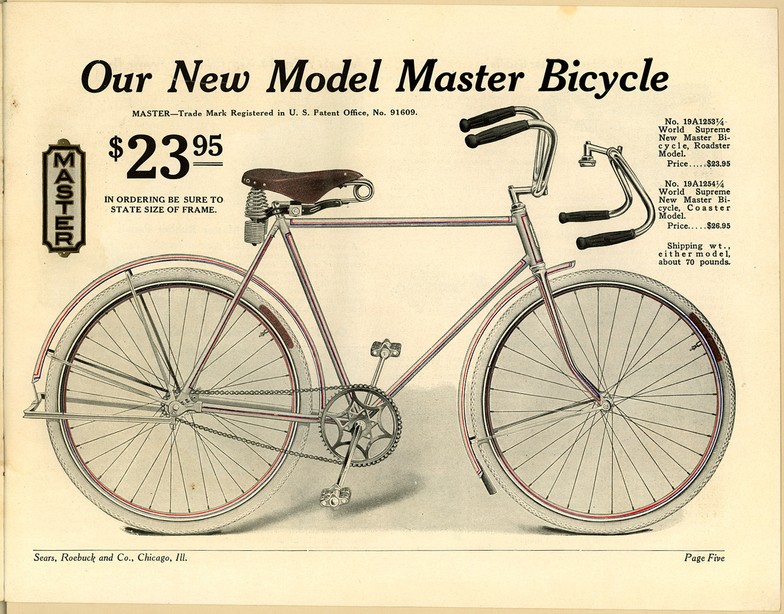This advertisement from Sears Roebuck and Company, located in Chicago, Illinois, appears on page 5 of their catalog and features a detailed illustration of an older brand bicycle. The title above the image reads "Our New Model Master Bicycle," with "Master Trademark registered in U.S. Patent Office number 91609" below it. The bike is priced at $23.95 for the roadster model, while the coaster model is listed at $26.95, with both models weighing approximately 70 pounds. The ad emphasizes the importance of specifying the frame size when ordering. The bicycle itself has a clean, traditional design with a standard saddle equipped with springs and options for either upwards or downwards handlebars, making it versatile. The ad is printed on slightly yellowed paper, giving it a vintage appearance.